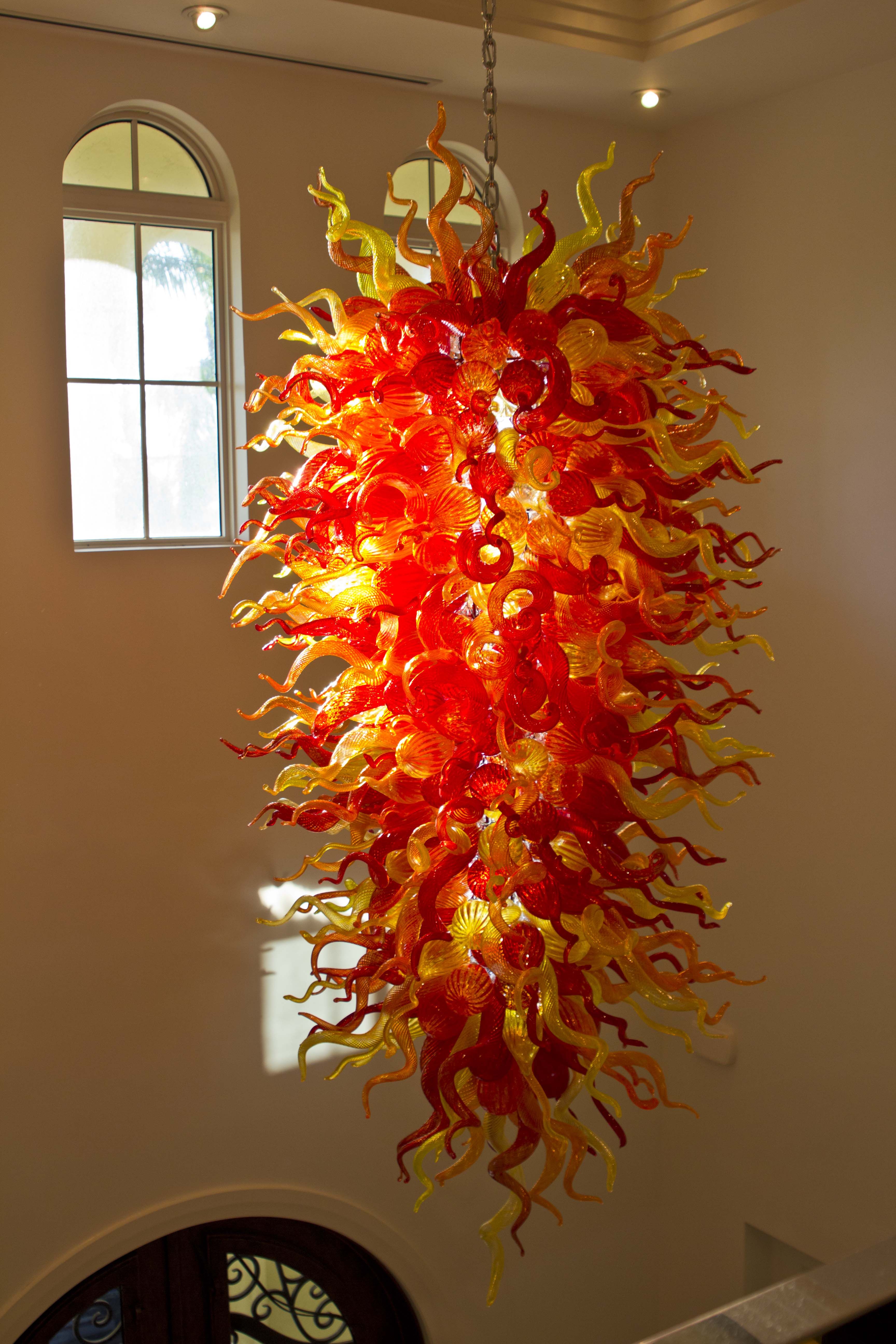The image is a digital photograph capturing a uniquely decorated chandelier with a striking design. The chandelier features numerous glass pieces tinted in red, orange, and yellow, arranged to resemble a vibrant fire. The glass pieces are meticulously crafted, creating an impressive pattern of light that reflects against the surrounding walls. The chandelier is elongated and hangs from a chain, making it the centerpiece of the room. Several lights are embedded within the chandelier, enhancing its fiery aesthetic. 

In the background, multiple windows with rounded tops can be seen, allowing natural light to filter into the room. These windows add a touch of elegance to the space. Additionally, the room contains a railing that complements the chandelier's design. The predominant colors in the image are yellow and red, with some hints of tan, white, and black, enriching the overall visual experience without any visible text to distract from the scene. The detailed craftsmanship and the interplay of colors make the chandelier a captivating focal point in the photograph.